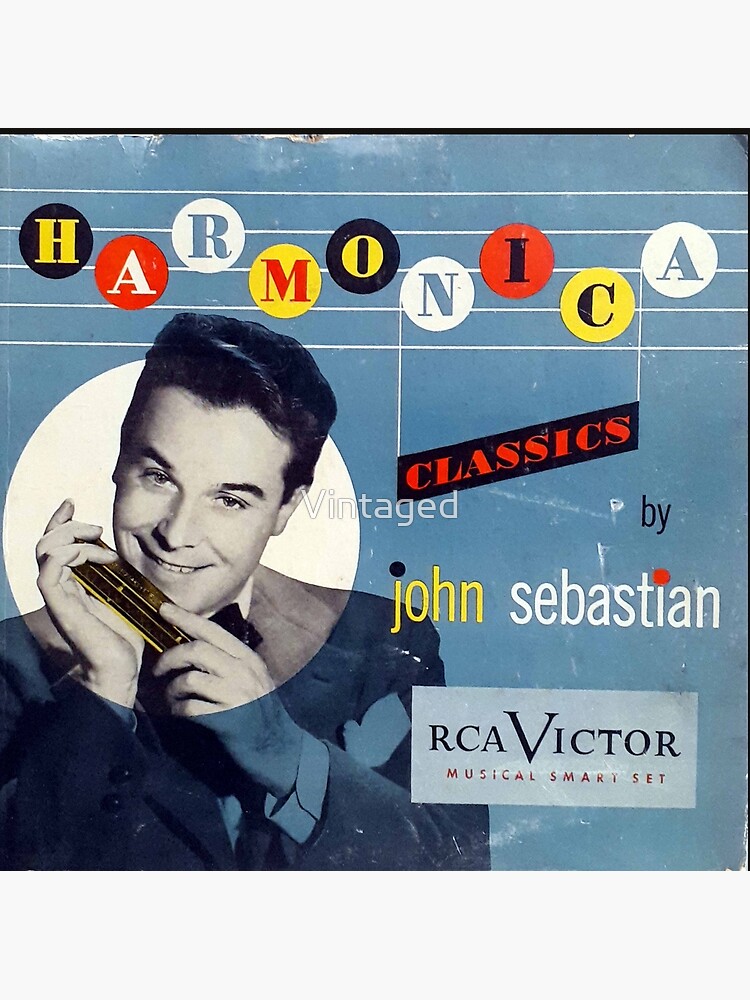This is a detailed visual description of a vintage album cover titled "Harmonica Classics" by John Sebastian from the RCA Victor Musical Smart Set. The background has a light blue hue, somewhat aged with visible rips and marks at the top, giving it a retro feel. At the top, the word "HARMONICA" is uniquely styled to resemble musical notes on a staff, with five horizontal lines extending across the cover. Each letter of the word "HARMONICA" is placed within a circle of varying colors: the letters and circles from left to right are a yellow H in a blue circle, a white A in an orange circle, a blue R in a white circle, a red M in a yellow circle, a yellow O in a blue circle, a blue N in a black circle, a black I in a white circle, followed by a black C and a final blue A in a white circle. Additionally, a bar connecting some of these notes is labeled "CLASSICS" in orange.

Positioned below the musical imagery, "by John Sebastian" is inscribed, featuring a blend of yellow and white hues with a black circle over the J and a red circle over the I. Accompanying this is a depiction of John Sebastian himself, presented in a black and white photograph that portrays him from the head to just above the chest level. Sebastian appears well-groomed with short brown hair styled in a classic 50s swoop. He is smiling warmly while playing a harmonica, which is spotlighted by a subtle white halo around his head and hands. The lower portion of the cover notes, "RCA Victor Musical Smart Set," providing further identification of the album's heritage. The entire composition conveys a charmingly nostalgic aesthetic, rich with musical and visual style.